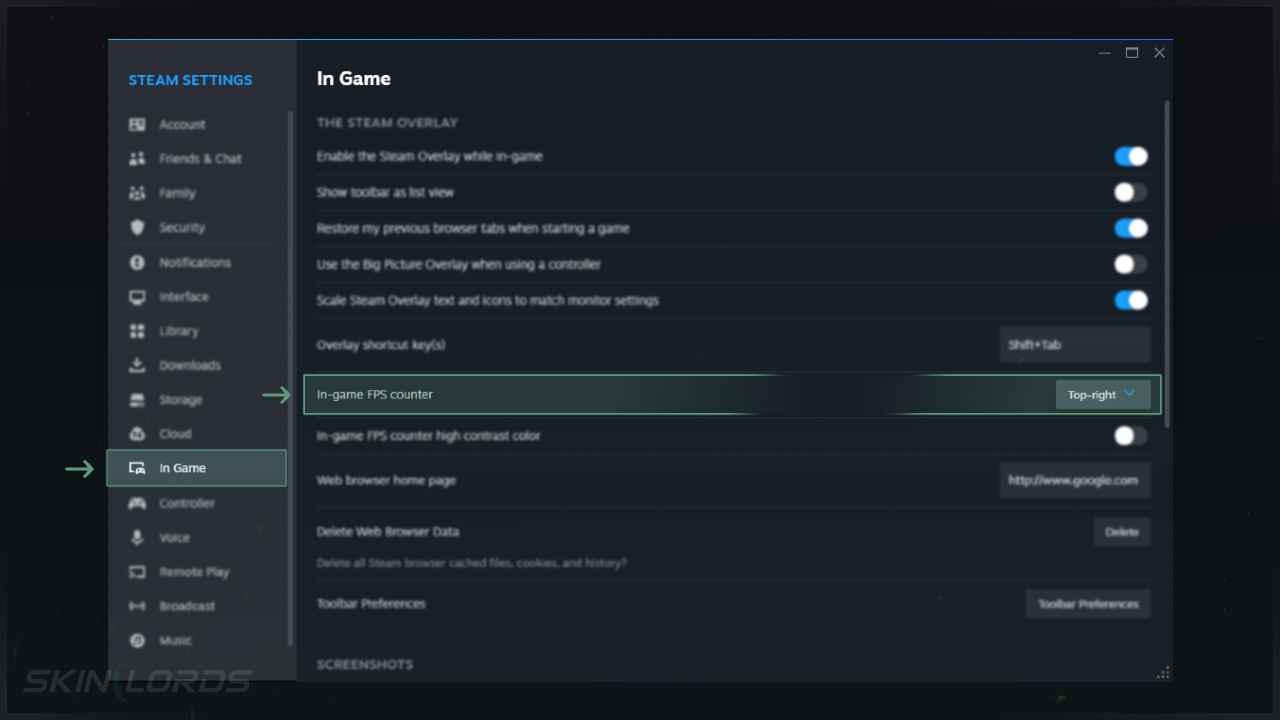The image appears to be a screenshot of the Steam Settings menu. In the upper left-hand corner, there is a blue header labeled "Steam Settings." Along the left-hand side of the window, a list of categories can be seen, though many are blurry. The readable categories include "Account," "Friends and Chat," "Family," "Security," "Notifications," "Interface," "Library," "Downloads," "Storage," "Cloud," "In-Game," "Controller," "Voice," "Remote Play," "Broadcast," and "Music." 

The "In-Game" category is highlighted in green, with a green arrow pointing towards it. In the more expansive right-hand column, at the top, it says "In-Game." Below this header, it mentions "Steam Overlay." Specific options under this section are hard to decipher due to the blurriness, but the highlighted sub-option, encased in a green box with an arrow, states "In-Game FPS Counter." To the right of this is a drop-down menu currently set to "Top Right."

The image shows various on/off toggle switches for different categories, indicating configurable settings. Though most of the options are unreadable, the word "Screenshots" is visible at the very bottom.